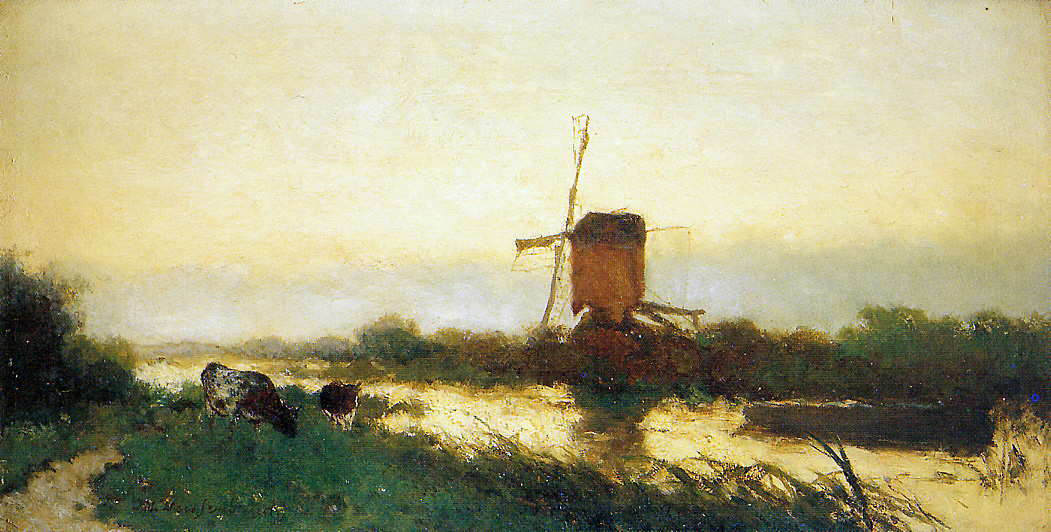This is an Impressionist oil painting of a serene, hazy landscape, wider than it is tall. Dominating the scene is a gently flowing river that meanders from the bottom right corner towards the upper left, partially obscured by a bush. On the left, a bit of land extends to the foreground, where two black and white cows graze on lush green grass. The background features an old Dutch windmill with tan walls and a dark brown roof, positioned in a side profile with its blades curving to the left. The sky above is a blend of muted yellowish tones, white, gray, and hints of blue, creating a smoky and smoggy atmosphere. A golden reflection of the light shimmers on the river, further adding to the painting's realistic yet ethereal quality. Surrounding the windmill, there are patches of tall grasses and bushes, with subtle beige and brown hues adding depth. Additionally, a faintly visible long brown boat sits near the windmill in the water, while two gray birds with black tails can be seen amidst the greenery.